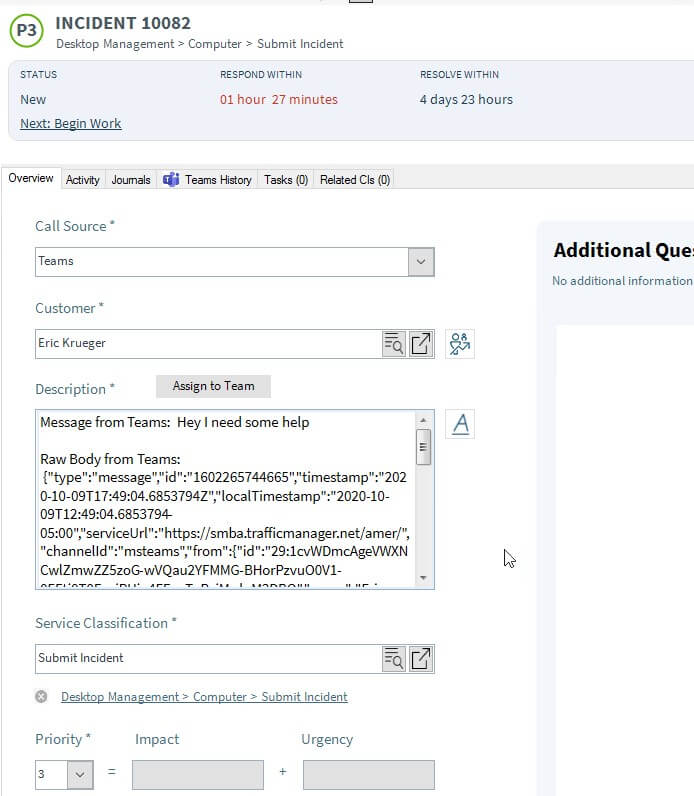The screenshot, set against a white background, prominently features a green circle in the upper left corner, containing the text "P3" in black. To its right, in bold black text, is the heading "Incident 10082". The caption beneath emphasizes "Complete that Desktop Management Computer Submit Incident."

The main content of the screenshot includes a light gray box with "Status New" written inside. Below it, further details are stipulated: "Next begin work," "Respond within 1 hour 27 minutes," and "Work within 4 days 23 hours."

Underneath these instructions is a form overview. It specifies a call source with a pull-down box set to "Teams" followed by a customer name field populated with "Eric Kruger." Adjacent to the description is an assignment button, and below it, a message reads, "Message from Teams: Hey, I need some help."

Further down, the form includes a "service classification" section, highlighting "Submit Incident" in the corresponding box.

This detailed description succinctly elaborates the information presented in the image, ensuring that each element is clearly identified and contextualized.